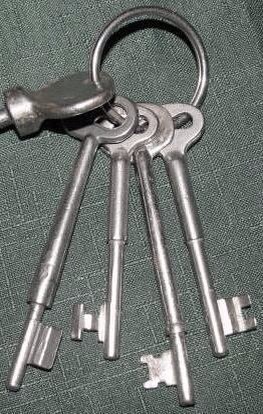On a dark grey-green fabric surface, there is a set of four vintage silver keys, each with a long body and a simple notched tip designed to unlock old-style doors. These metallic silver keys are clustered together on a large circular key holder. The photograph is an extreme close-up, capturing the keys in great detail but obscuring any surrounding environment. One key extends horizontally from the key ring, with its edge cropped by the image, while the other three keys point downward at slight angles to the left and right. The key ring casts a faint shadow at the top of the image, and attached to the ring is another silver item, possibly part of a key, but it's slightly out of focus and difficult to identify. The fabric beneath appears textured, adding depth to the composition, and the light source seems to be coming from above, casting a subtle shine on the tips of the keys and enhancing their metallic sheen.